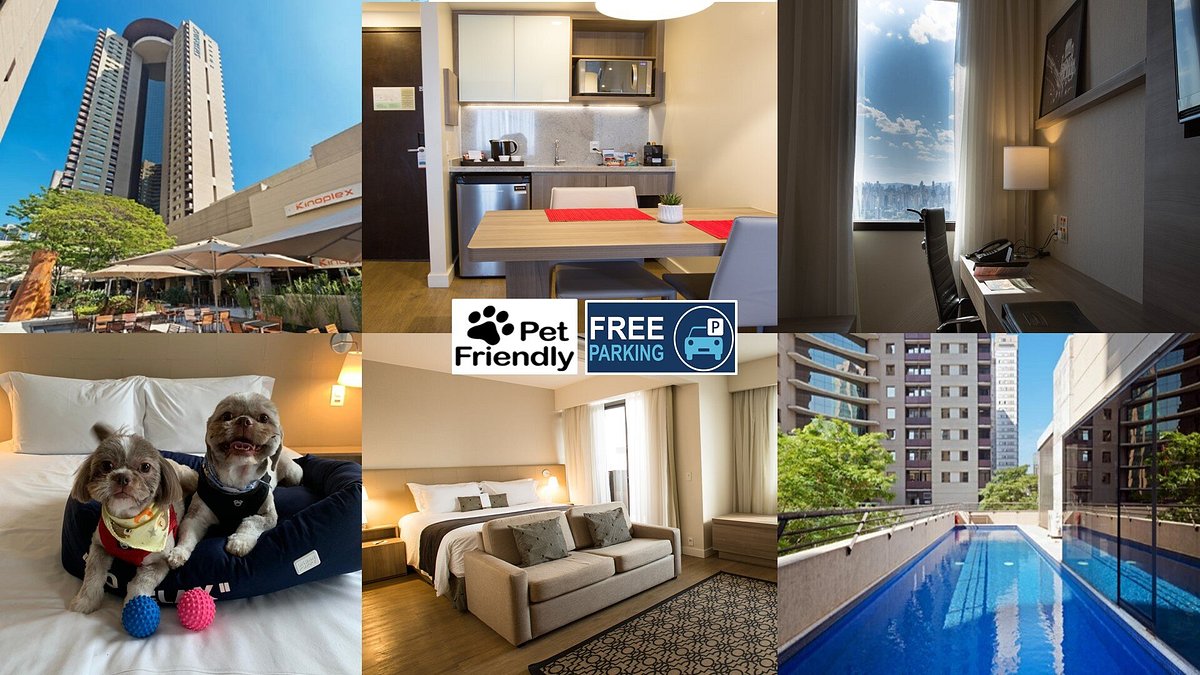The image is a detailed collage comprised of six photographs, arranged in two rows of three. Centrally positioned between these images is a white rectangle with black text reading "Pet Friendly," flanked by a black paw print, and a navy rectangle with a white outline stating "Free Parking," including an icon of a car and a “P.”

In the upper left corner, the image depicts a tall hotel building surrounded by trees and a small building to the right, with an outdoor seating area featuring umbrellas in the foreground. The central top image shows a kitchenette and dining area within a hotel room, identifiable by a table and chairs. To the upper right, there's a workspace area with a desk, chair, and table lamp positioned near a window adorned with white curtains.

The bottom left photograph highlights a white bed with two small dogs playing on it, accompanied by a blue cushion and colorful balls. The central bottom image presents a wider view of the bedroom, displaying the bed, a gray sofa with cushions in front of it, hardwood flooring, and windows to the right. The bottom right image captures an outdoor pool, bordered by stone fencing and surrounded by tall buildings and trees.